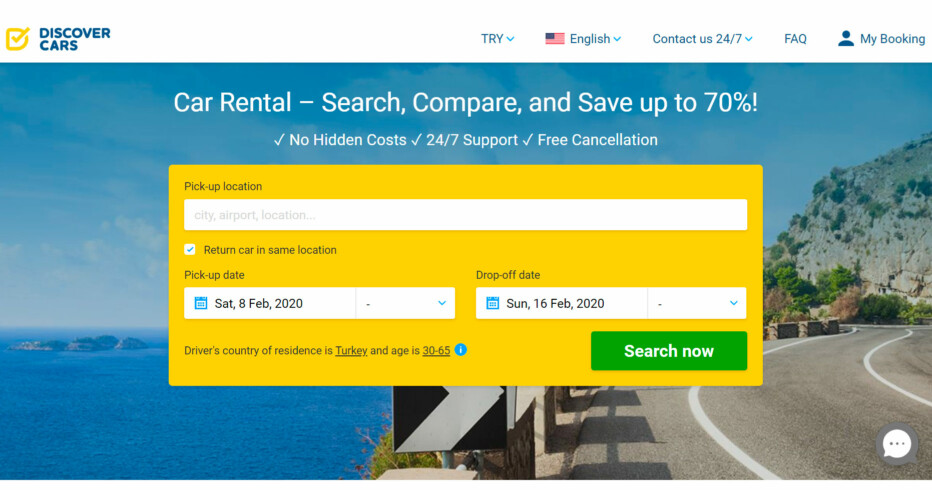This image shows the "Discover Cars" webpage, prominently branded with its blue logo and yellow 'D' icon at the top left. Across the top right, there are several interactive tabs, including options to change the language ('Try English'), contact support ('Contact Us 24x7'), access the FAQ, and click through to 'Profile' and 'My Booking'. 

In the center of the page, a bold headline in white text announces: "Car Rental: Search, compare and save up to 70%. No hidden cost. 24x7 support. Free cancellation." Below this, a search form is visible that features fields for 'Pickup Location' and an interactive checkbox labeled 'Return Car to Same Location.' Accompanying date fields for 'Pickup Date' and 'Drop Off Date' also appear. 

Towards the bottom left, the website states the user's country of residence as Turkey and age range as 30-65. On the bottom right, a prominent green button labeled 'Search Now' invites users to initiate their search.

The background of the page is a vibrant yellow, contrasting with the central content. Along the bottom, a scenic image serves as a backdrop: a serene blue lake on the left, a winding grey road with white lines on the right that curves to the right, bordered by rocky mountains with patches of dark green trees.